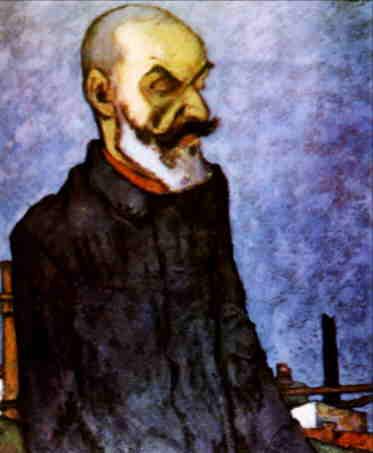This detailed painting depicts an older man with a prominent black mustache and a white beard, facing slightly forward and to his right. His receded hairline reveals sparse, gray hair, and his balding head emphasizes his age. He has large black eyebrows and a few facial spots, adding character to his face. The man's attire includes a red shirt partially covered by a black coat or robe. The background features hues of blue and purple, suggesting a watercolor technique. To his right, there's an ambiguous wooden object, possibly a table, chair, or barrel, along with some indistinct items that contribute to the scene's setting. The man appears to be holding an unidentified object in his left hand, which could be a knife or a cross, giving an impression of contemplation or meditation. This richly detailed composition evokes curiosity and invites viewers to imagine the story behind the serene yet enigmatic figure.